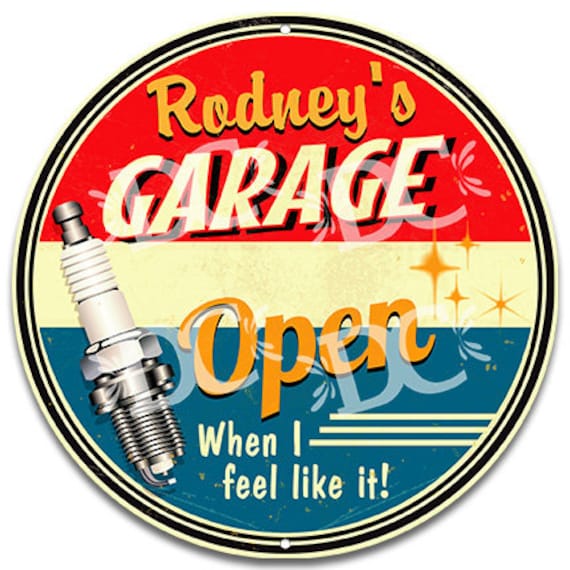The image depicts a circular metal sign against a white background. The sign is bordered by a beige outer ring, followed by alternating black and white striped borders. The top section of the sign features a red background with the text "Rodney's Garage" prominently displayed; "Rodney's" is in orange letters, while "Garage" is in block-style white letters with a red outline. The middle section of the sign has a light beige band that runs horizontally across, adorned with some gold starburst shapes. In the lower portion, a blue background houses the word "Open" in gold letters, partially extending to the beige section above. Directly below, it reads "When I feel like it!" in white letters. Additionally, the left side of the sign displays an image of a spark plug, extending from the bottom blue area up into the red top. There are also digital watermarks featuring the letters "DC" with splash marks, twice over the red and twice over the blue sections. The sign appears to have mounting holes at the top and bottom for attaching it to a wall.